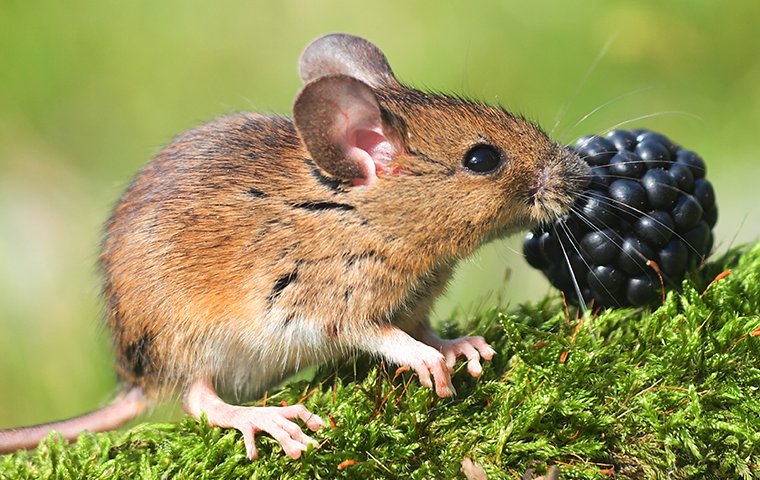This outdoor daytime photograph captures a close-up view of a small, brown mouse nestled atop a vibrant green, fluffy fir or fern branch. The mouse, positioned in the lower left-hand corner, faces the right-hand side of the image, where its hairless pink tail extends off-screen. Its pinkish feet and hands, black eyes, long white whiskers, and small pink ears are clearly visible. The mouse's nose rests on a plump, full blackberry situated just in front of it. Behind the mouse, the background is blurred into a greenish hue, devoid of any distinct details, creating a soft focus that emphasizes the mouse's charming details and the vividness of the foliage and fruit.